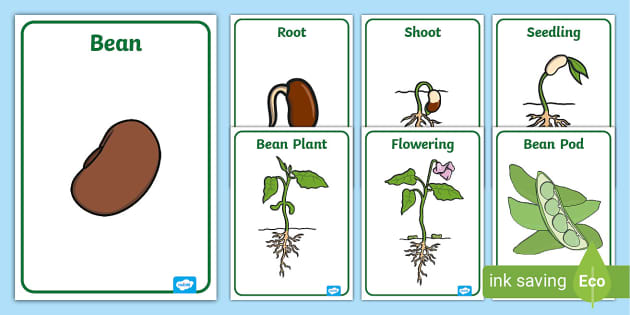This educational illustration presents a detailed depiction of the life cycle of a bean plant. It begins with an individual brown bean labeled "Bean" and progresses through the successive stages: "Root," where the bean develops white roots; "Shoot," where green shoots start to emerge; followed by "Seedling." The sequence continues with an image of a fully formed "Bean Plant," complete with green leaves, and then to the "Flowering" stage, showcasing a purplish flower. The final stage illustrates the "Pod," displaying green pods containing new beans. 

The illustration is framed with a green border set against a white background, and the text labels throughout are in green. A logo in the bottom right corner reads "Ink Saving Eco," highlighting the eco-friendly theme. The overall color scheme focuses on the natural colors of the bean plant: the brown of the beans, white roots, green shoots and leaves, and purple flower, maintaining an informative and visually appealing graphic.